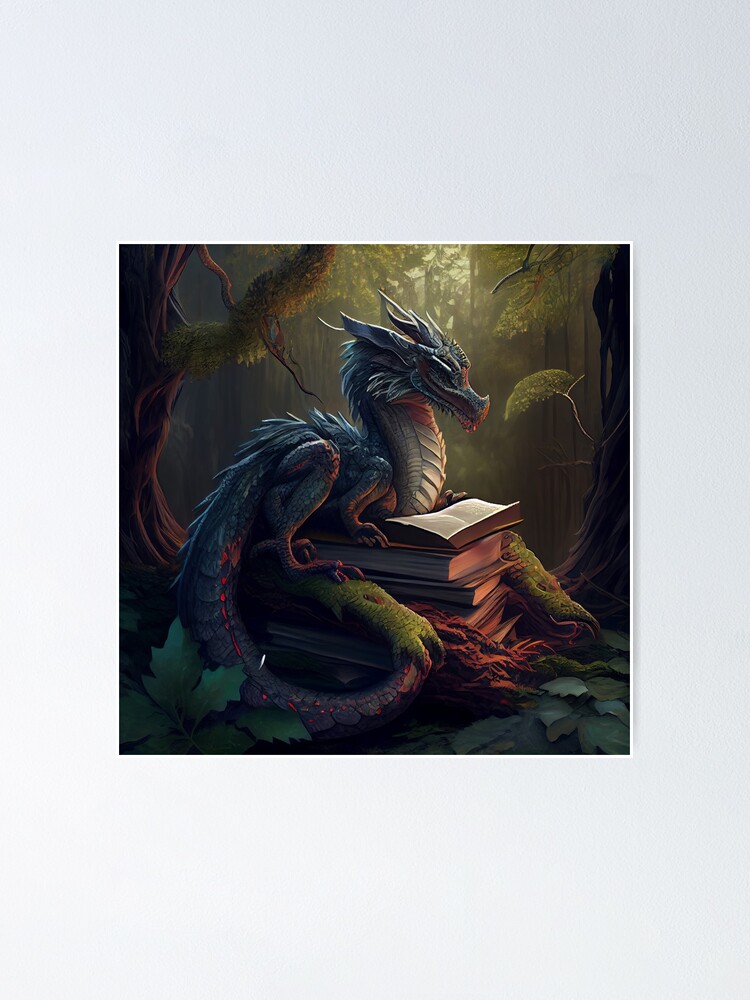This detailed computer graphic artwork portrays a majestic dragon perched on a stack of about five or six books in the heart of a sun-dappled fantasy woodland. The dragon, covered in shimmering blue scales with accents of red, is the focal point of the image. Its two powerful feet rest securely on the books, while its side profile reveals it fixated on an open book, suggesting it's deeply engrossed in reading. The creature's belly and neck areas feature a transition to white scales, adding to its intricate design. The lush forest background sets a serene atmosphere: ivy leaves spread beneath the dragon and the books, while sunbeams penetrate the forest canopy, casting a magical glow on the scene. The left side of the image is dominated by a tall tree draped in moss, with more trees fading into a green-hued distance. This enchanting artwork is displayed as a square piece encased in a large white rectangular border, enhancing its presentation.